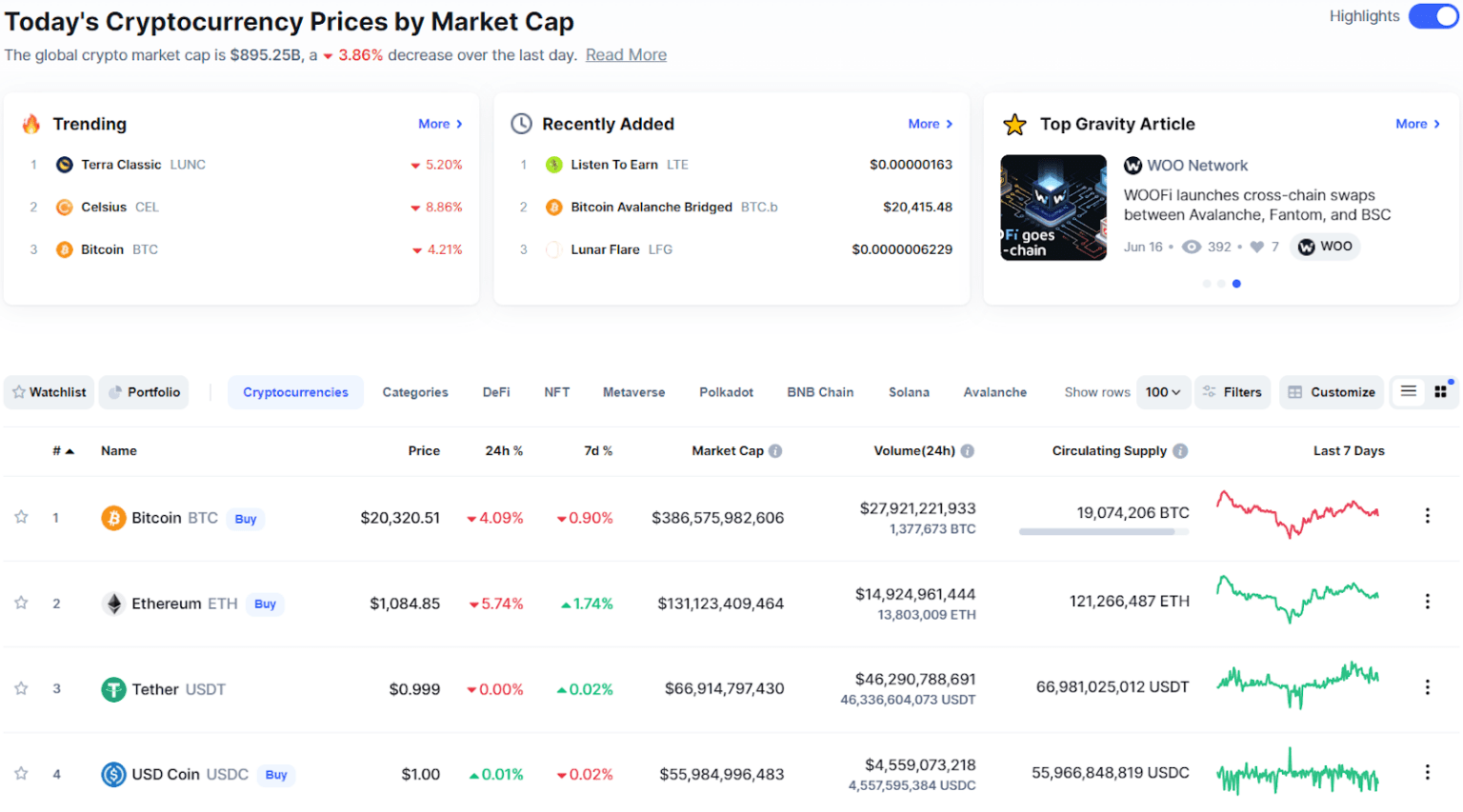### Detailed Description of Cryptocurrency Trends by Market Cap

The image showcases detailed trends in the cryptocurrency market, focusing on various metrics such as market capitalization, price movements, and trending cryptocurrencies.

**Main Panel:**
1. **Global Overview:**
   - *Title:* Cryptocurrency Trends by Market Cap.
   - *Statistic:* The global crypto market cap stands at $895.25 billion, having decreased by 3.86% over the last day.

2. **Trending Cryptocurrencies:**
   - *Highlighted Section (Top Right):* The 'Highlights' section is toggled on, showing the top trending cryptocurrencies.
     - **1. Terra Classic (LUNC):** Down by 5.2%.
     - **2. Celsius (CEL):** Down by 8.86%.
     - **3. Bitcoin (BTC):** Down by 4.21%.
   - *Additional Features:* There's a "Read More" link and a "More" button indicated by a greater-than sign for further details.

3. **Recently Added Cryptocurrencies:**
   - Displayed with a clock icon and a "More" button (greater-than sign).
     - **1. Listen to Earn (LTE):** Priced at .000000163.
     - **2. Bitcoin Avalanche Bridged BTC (BTC.b):** Priced at $20,415.48.
     - **3. Lunar Flare (LFG):** Priced at .0000006229.

4. **Top Gravity Article:**
   - *Article Title:* "Woo Network: WooFi launches cross-chain swaps between Avalanche, Phantom, and BSC."
   - *Date:* June 16th.
   - *Engagement Metrics:* 392 views and 7 likes.
   - *Navigation:* Three navigation circles, with the third circle highlighted in blue.

**Lower Panels:**
1. **Navigation and Filtering Options:**
   - *Categories:* Watchlist, Portfolio, Cryptocurrencies, Categories (DeFi, NFT, Metaverse, Polkadot, BNB chain, Solana, Avalanche).
   - *Default Selection:* Cryptocurrencies.
   - *Display Options:* Show rows up to 100, with filters for customization. The list can be viewed in different formats (indicated by three lines and four squares icons), currently viewed line by line.

2. **Detailed Cryptocurrency Table:**
   - **1. Bitcoin (BTC):**
     - *Indicator:* Starred as the top entry.
     - *Price:* $20,320.51.
     - *24-Hour Performance:* Down 4.09%.
     - *7-Day Performance:* Down 0.90%.
     - *Market Cap:* $386,575,982,606.
     - *24-Hour Volume:* $27,921,221,933.
     - *Circulating Supply:* 19,074,206 bitcoins.
     - *Price Trend:* Depicted with a red graph for the past seven days.
   - This trend follows for other cryptocurrencies such as Ethereum, Tether, and USD Coin.

Overall, the image provides a comprehensive view of the cryptocurrency market, including its top performers, newly added coins, and detailed statistics for major cryptocurrencies.